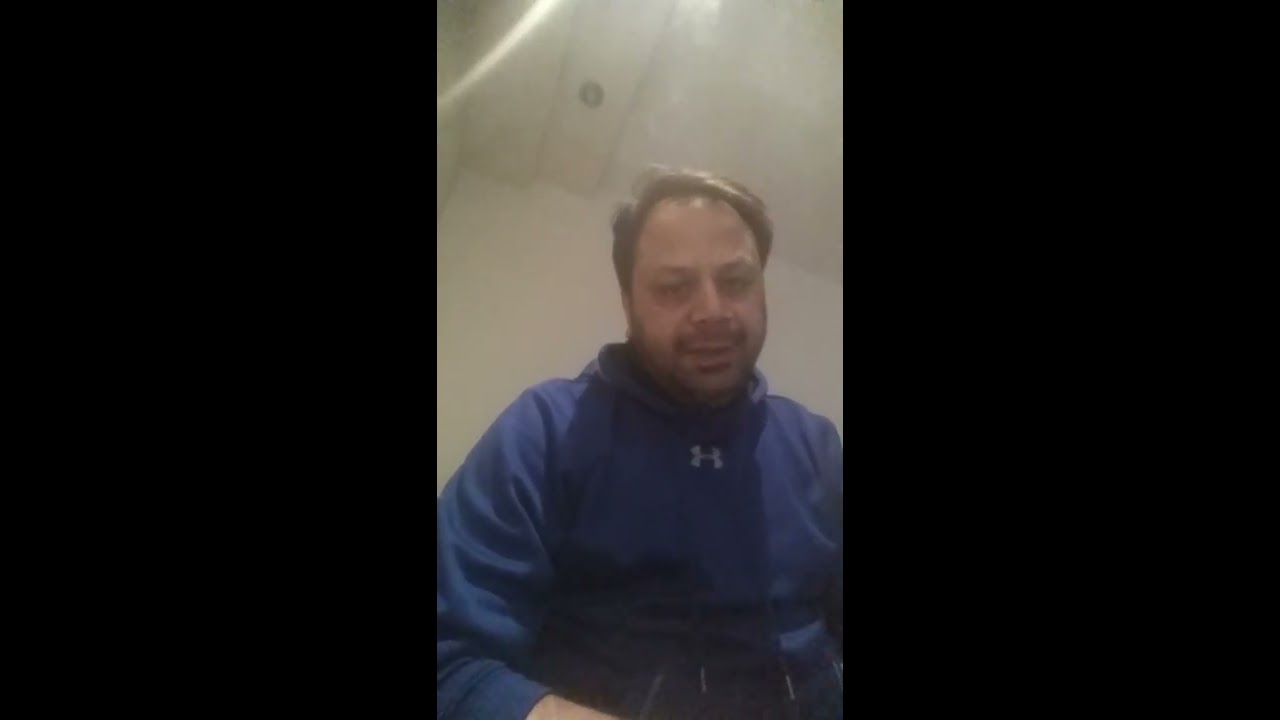The image features a light-skinned Indian man with brown hair and a lightly shaved beard, sitting and looking directly at the camera, likely taking a selfie. He is wearing a navy blue Under Armour pullover hoodie with a hood attached and strings hanging down. The background shows a white or light tan room with a ceiling made of square tiles, and a round metal light fixture is visible above him. The photo, which is somewhat fuzzy and of low resolution, is divided into three vertical sections, with the middle section displaying the man's image while the first and third sections are completely black. The man is centered in the image, seen from his stomach upward. There is not much detail indicating the specific location of the room, making it appear quite plain.